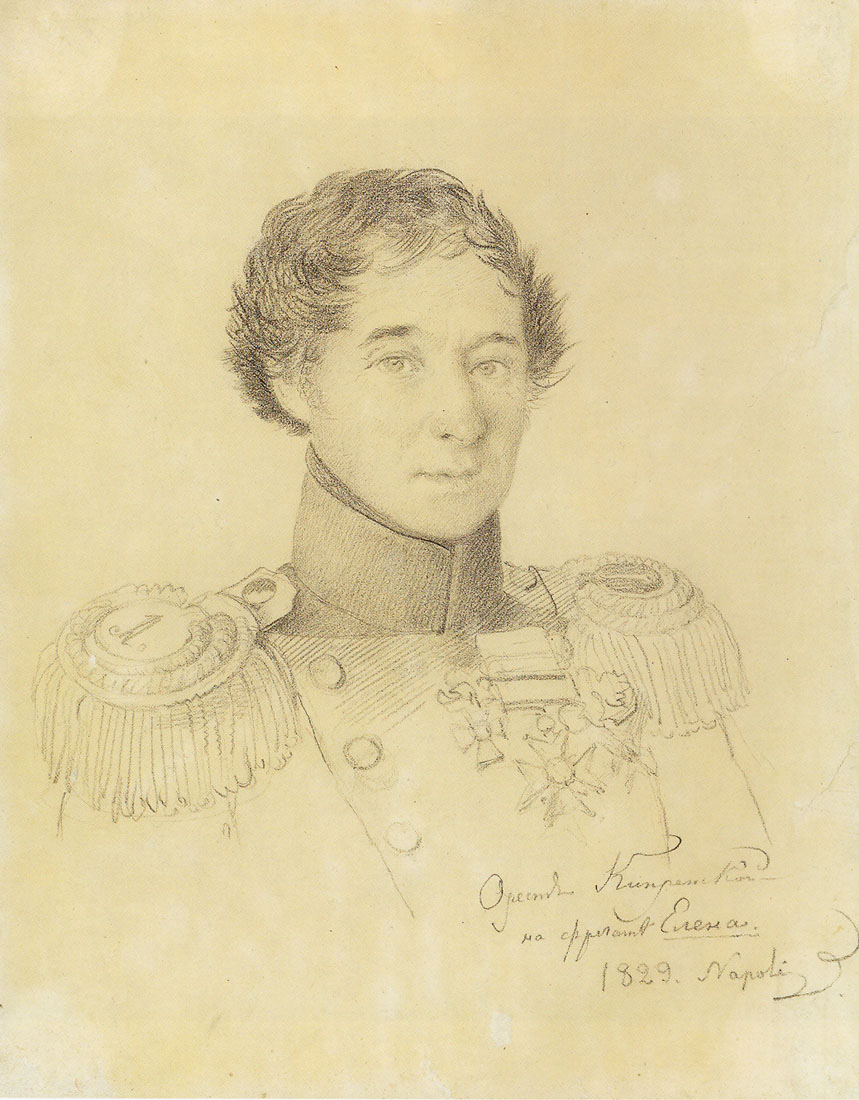This detailed sketch, possibly a pencil drawing or an engraving, depicts a 19th-century army officer, potentially from the Napoleonic era, given the date "1829" and the inscription "Napoli" at the bottom, which suggests a connection to Naples, Italy. The subject appears to be in his early 30s with dark, short, bushy hair and expressive eyes gazing towards the front, effectively engaging the viewer. He is dressed in a traditional military uniform adorned with epaulets that feature a brush-like embellishment and several medals on his chest. The right side of his uniform is marked by three prominent buttons. The background is a soft beige, reminiscent of watercolor, although primarily black ink is used on the brown paper. The text at the bottom is written in Italian and, while hard to decipher fully, reinforces the historical context of the figure portrayed.